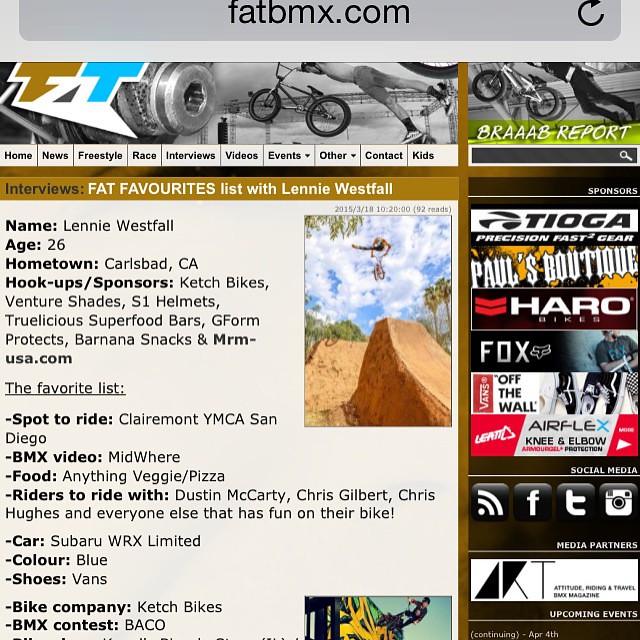The image is a detailed screenshot of a BMX website viewed on a smartphone, probably an iPhone, with the URL fatbmx.com visible along with a refresh symbol. The website's banner features a logo and an eye-catching picture of a BMX rider performing a superman trick on his bike. At the top of the page, the heading reads "Interview FAT Favorites List with Lenny Westfall," revealing it to be an interview segment. The interview showcases details about Lenny Westfall, including his age (25/26) and hometown (Carlsbad, California). His listed sponsors are Ketch Bikes, Venture Shades, S1 Helmets, Truelicious Superfood Bars, G-Form Protects, Banana Snacks, and MRMUSA.com. The page documents his favorite riding spots such as Claremont YMCA and San Diego BMX; his preferred video as Midwear; and his favorite food, veggie pizza. Moreover, it mentions other riders he enjoys biking with, specifically Dustin McCarty, Chris Gilbert, and Chris Hughes. Additional personal details include his car, a blue Subaru WRX Limited, his preference for Vans shoes, and his bike company, Ketch Bikes. The background of the page includes various colors such as gray, orange, light brown, green, red, yellow, cream, blue, silver, and teal. There are also advertisements positioned to the right side, likely relating to BMX products and gear.